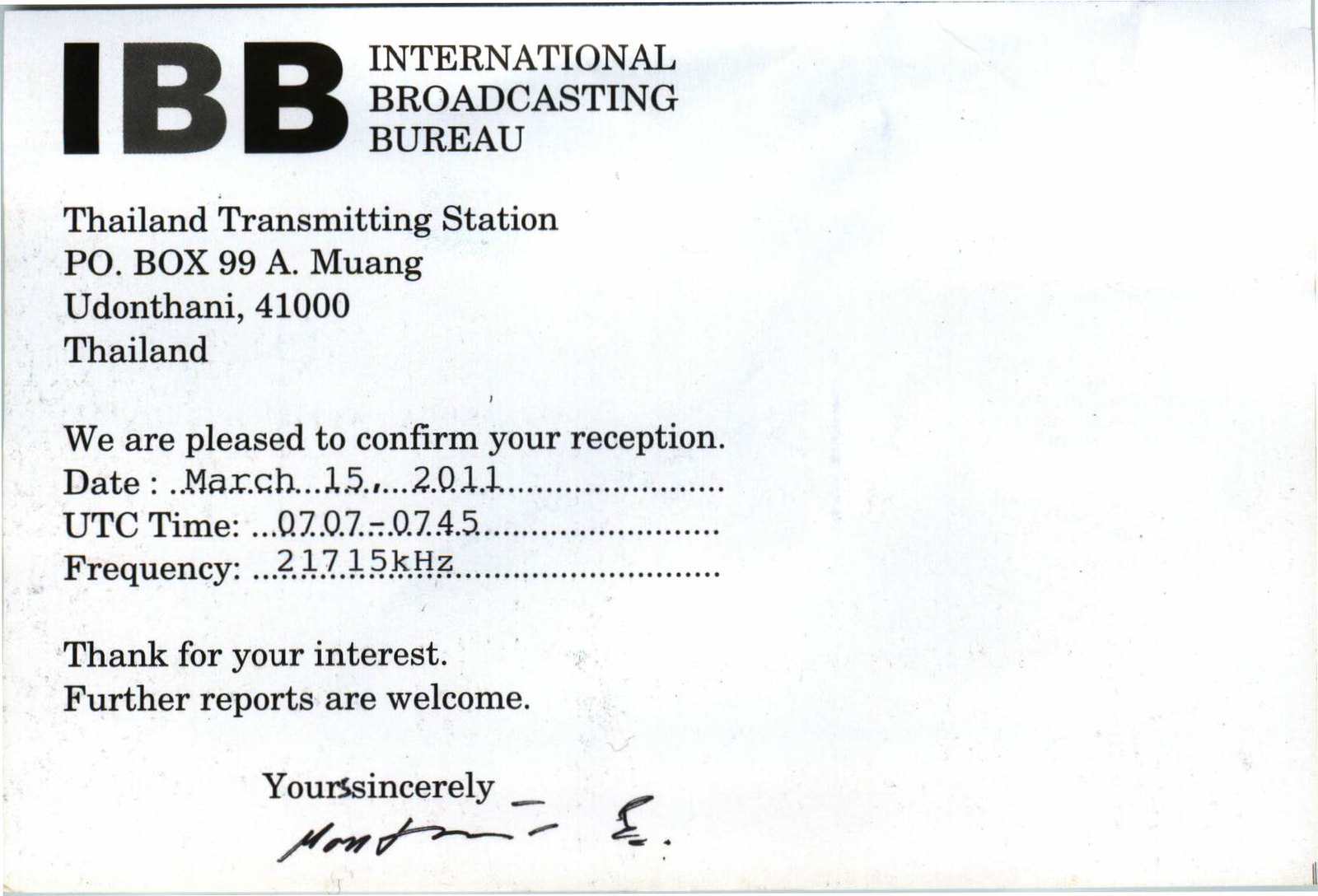The image displays a slightly aged confirmation document from the International Broadcasting Bureau (IBB), prominently featuring large block letters "IBB" at the top left corner, with the words "International Broadcasting Bureau" stacked vertically to the right. Below this header, in a serif font resembling Times New Roman, the document specifies the Thailand Transmitting Station, located at PO Box 99A, Muang, Udon Thani, 41000, Thailand. It confirms reception on March 15th, 2011, in the UTC time frame of 0707-0745, on the frequency band of 21715 kHz, written in a courier typewriter style font. The text concludes with a polite note, thanking the recipient for their interest and encouraging further reports, followed by "Yours sincerely" and a black signature that appears somewhat illegible but seems to begin with "mont." The document shows minor imperfections such as blotches, indicative of it being a photocopy, and slight wrinkles in the top right corner, suggesting the paper is not brand new. All text is aligned to the left, leaving the right side nearly blank.